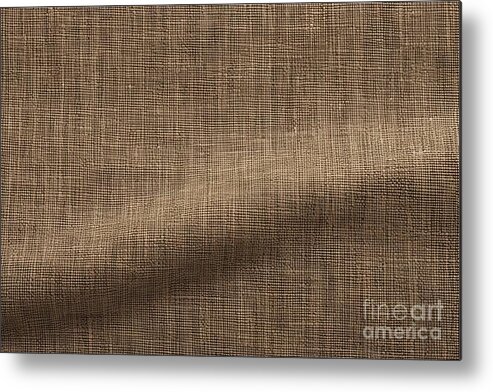The photograph captures a three-dimensional, rectangular piece of textile, resembling woven tweed or burlap, featuring an intricate pattern of horizontal and vertical stripes in varying shades of brown and tan. The fabric displays a noticeable, slightly diagonal wrinkle or lift, suggesting it wasn’t completely pressed flat, casting subtle shadows that emphasize its texture and depth. The background of the image is a white surface, enhancing the textile's earthy tones. In the bottom right corner, a watermark reading "Fine Art America" appears, with the word "Fine" in a thin, fine font and "Art America" in thicker letters, slightly standing out against the fabric’s texture.